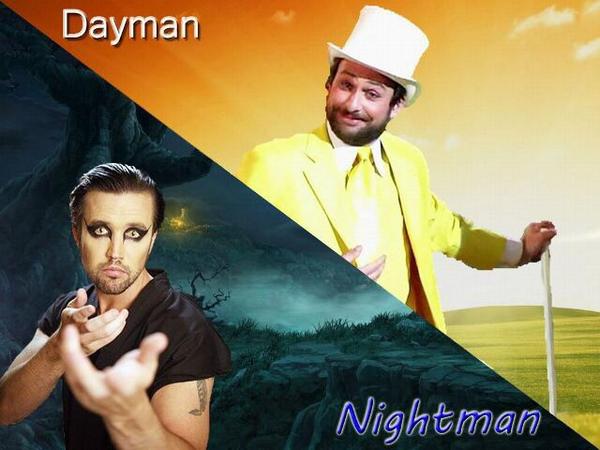The image is a split rectangle, divided diagonally from the upper left to the lower right corner, showcasing two iconic characters from "It's Always Sunny in Philadelphia," Dayman and Nightman. In the upper right section, against a bright landscape with an orange sky, grassy fields, and low hills, stands Charlie Day as Dayman. He is dressed in a yellow suit with a yellow tie, a white shirt, and a white top hat. He is smiling, with his left hand holding a white cane and his other hand resting on his suit jacket. The word "Dayman" appears in white letters in the upper left part of this section. In contrast, the lower left section features Rob McElhenney as Nightman, set against a dark, eerie background with mist, an old tree, a candle, and dark rocks, evoking a cemetery-like environment. Nightman is characterized by black eyeliner, slicked-back hair, a dark goatee, and a black short-sleeved shirt with a tattoo visible on his left bicep. He is looking directly at the camera while reaching out with his hands. The word "Nightman" appears in blue letters at the lower right corner of this section.